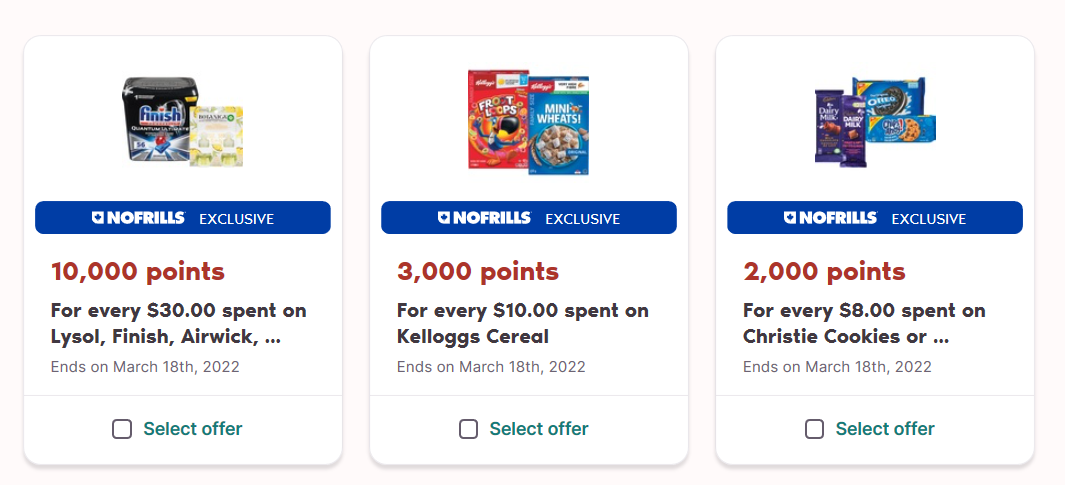The image features a light blue background with three prominent white boxes. 

1. The first box contains a black rectangle labeled "Finish" beside a small yellow and white package. Additionally, there is a purple banner stating, "No Frills Exclusive: 10,000 points for every $30 spent on Lysol, Finish, or Airwick," along with an option labeled "Select Offer" at the bottom.

2. In the second box, there are packages of Froot Loops in a red box and Mini-Wheats in a blue box. A purple banner informs, "No Frills Exclusive: 3,000 points for every $10 spent on Kellogg's cereals," applicable until March 18th, 2022. Below this is also a "Select Offer" option.

3. The third box showcases Oreo cookies, Chips Ahoy, and two small bags of other snacks. Another purple banner announces, "No Frills Exclusive: 2,000 points for every $8 spent on Kristy Cookies," valid until March 18th, 2022, with a "Select Offer" box at the bottom.

This detailed promotional image highlights various products and their respective exclusive points offers at No Frills.